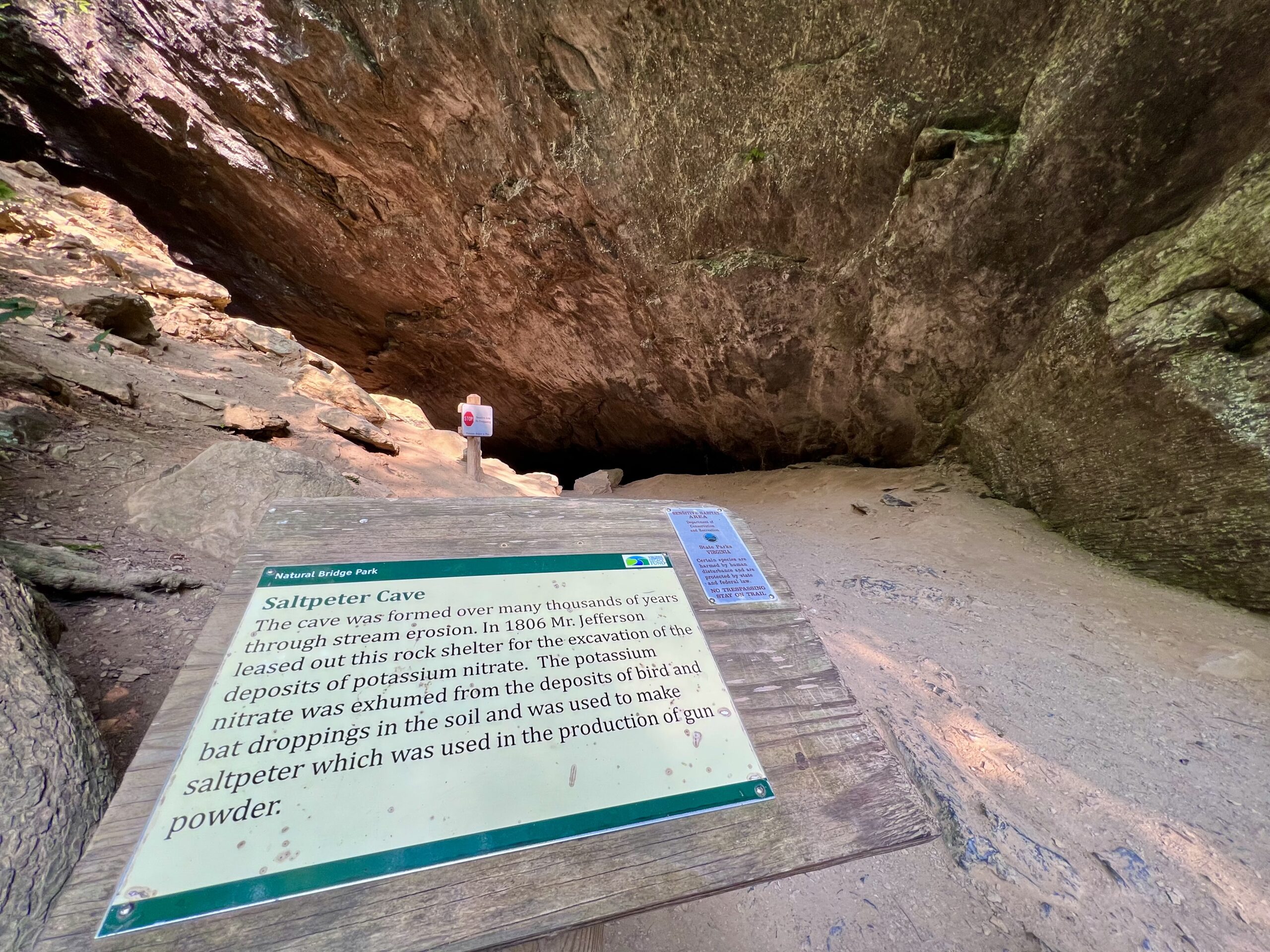The photograph captures the entrance of Saltpeter Cave, surrounded by gray and brown rock formations. The cave, which was formed over thousands of years through stream erosion, has an opening that sits at the intersection of two large rock faces. In the foreground, there is a prominent wooden podium, which features an informational plaque with details about the cave. The plaque has a teal border on the top and bottom, with "National Bridge Park" written in white lettering on the top section. Below that, "Saltpeter Cave" is displayed in bold black lettering, followed by text explaining that in 1806, Mr. Jefferson leased the cave for the excavation of potassium nitrate from the deposits of bird and bat droppings, which was used to produce gunpowder. Additionally, the background features a small sign with a red circle near the entrance, though its details are not legible from the photograph. The image vividly combines the natural aspects of the cave's entrance with historical information presented in the foreground.